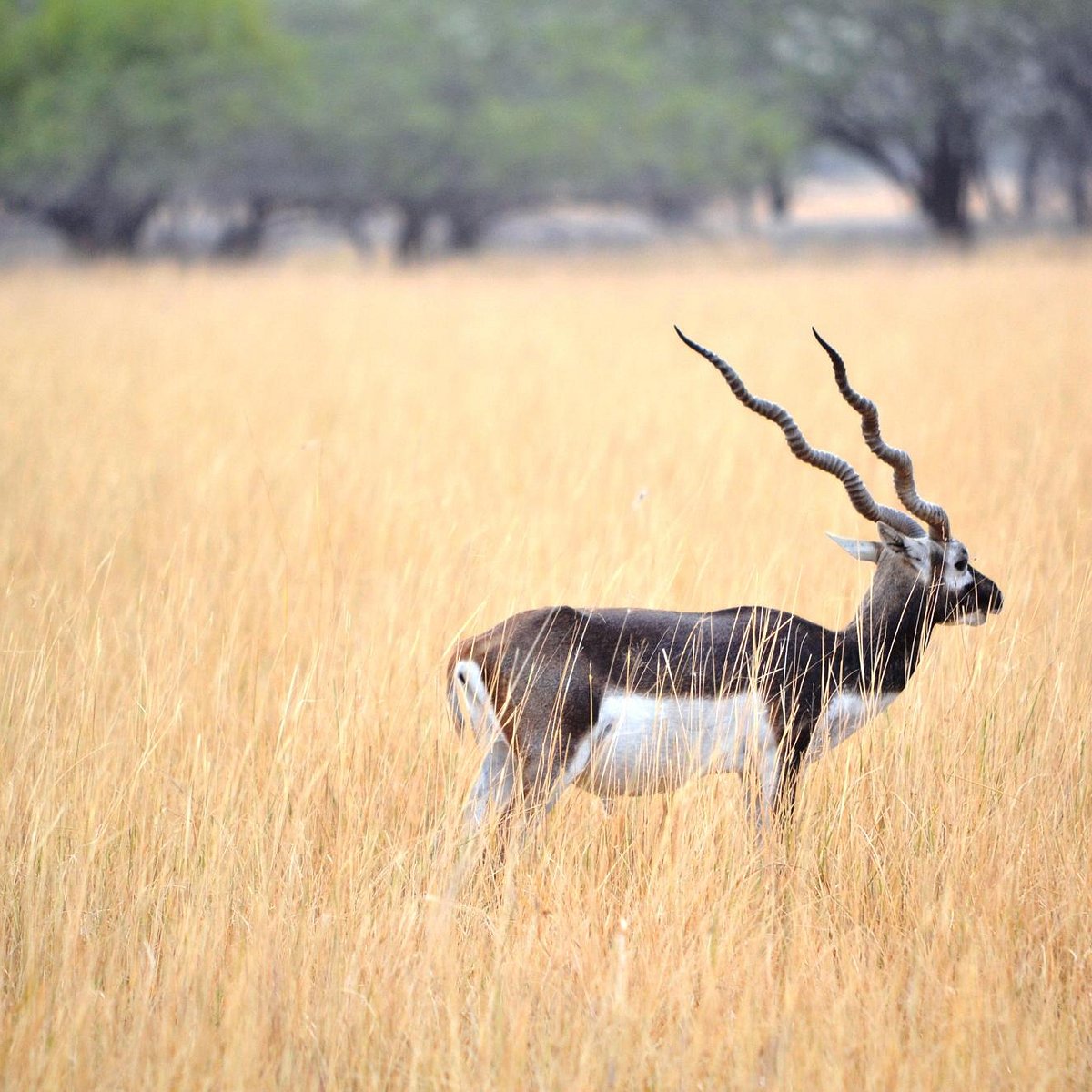In this nature photograph, an eland antelope stands gracefully in a large, uniform field of tall, light brown grass, which extends up to its waist. The eland, looking towards the right side of the image, is characterized by its striking coloration: a white belly contrasting with a dark brown back, neck, and hindquarters. Its head is adorned with two prominent, spiraled horns that are both long and sharp. The background features a blurred outline of expansive trees, enhancing the depth of field and adding a secluded, natural ambiance to the scene. The overall composition highlights the solitary majesty of the eland within its serene, natural habitat.